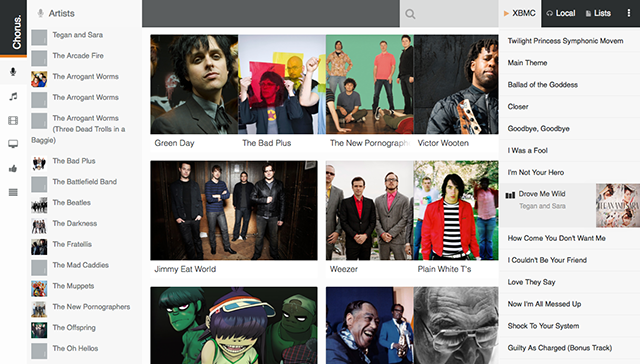This image depicts a webpage with a distinct layout and various elements. In the upper left corner, the text "chorus" is written twice, once in what seems to be a dot-separated web address as "chorus dot c-h-o-r-u-s dot." Directly below this, on the left side, there is a microphone icon. Beneath the microphone, there's an orange vertical line set within a black tab, and at the bottom, the word "chorus" is written in white, vertically aligned.

To the right of these icons, there's a sequence of additional symbols including a music note, film reel, monitor, thumbs up, and four horizontal lines stacked. Adjacent to these symbols to the right, several artist names are listed: Tegan and Sara, Arcade Fire, The Arrogant Worms (repeated), Three Dead Trolls in a Baggie, The Bad Plus, The Battlefield Band, The Beatles, The Darkness, The Fratellis (possibly misspelled as F R A T O L L I S), The Mud Codys, The Muppets, The New Pornographers (possibly misspelled as the new photographers), The Offspring, and The Oh Hellos.

Below this list, there’s a gallery of photographs associated with various bands and artists. Labeled images include Green Day, The Bad Plus, The New Pornographers (possibly misspelled), Victor Wooten, Jimmy Eat World, Weezer, and Plain White T's (referred to as "paying white tees"). Additional photographs are visible but not labeled.